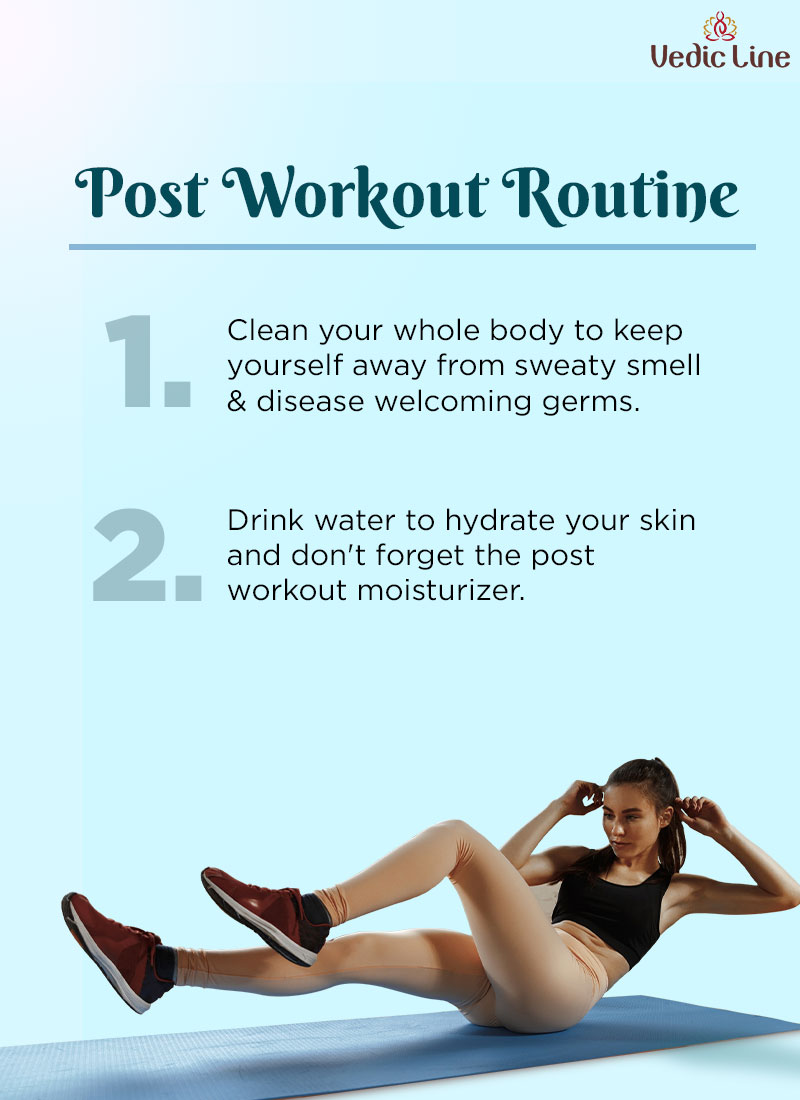The image is a detailed informational poster in portrait orientation, featuring a light blue-green gradient background. In the upper left corner, a white light fades as it moves downward, while the upper right corner hosts a red or possibly brown drawing of a person in a lotus pose, accompanied by the text "Vedic Line." Centered about a third of the way down, the headline "Post-Workout Routine" is written in a teal, slightly script font and underlined in blue. Below the headline are two numbered instructions in blue text: 

1. "Clean your whole body to keep yourself away from sweaty smell and disease-welcoming germs."
2. "Drink water to hydrate your skin and don't forget the post-workout moisturizer."

At the bottom, there's a horizontal photograph occupying the bottom quarter of the poster, featuring a young woman of Caucasian descent, dressed in beige leotards, a black halter top, and black sneakers. She is lying on a blue yoga mat, positioned as if performing a bicycle crunch with her hands behind her head and knees drawn towards her chest. The overall aesthetic combines photographic realism with graphic design and informative typography.